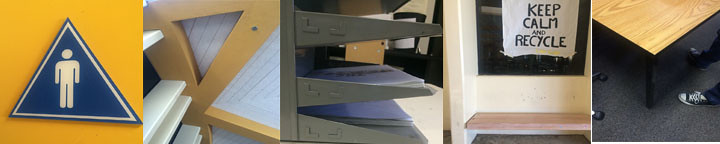The image consists of five square pictures arranged side-by-side. The first picture features a yellow background with a blue triangle outlined in white, containing a white silhouette of a man, resembling a bathroom sign. The second picture shows an ambiguous structure with brown wood and white paneling against a bluish-gray background, including a triangle cut into the wood. The third picture depicts three dark brown, almost black, metal shelves typically used for organizing papers on a desk. The fourth picture contains a black and white sign reading "Keep Calm and Recycle," seemingly placed on a wall or window, with a plastic bench visible nearby. The fifth and final picture captures the corner of a wooden desk with black legs on a commercial carpet, including a visible person's shoe on the ground.